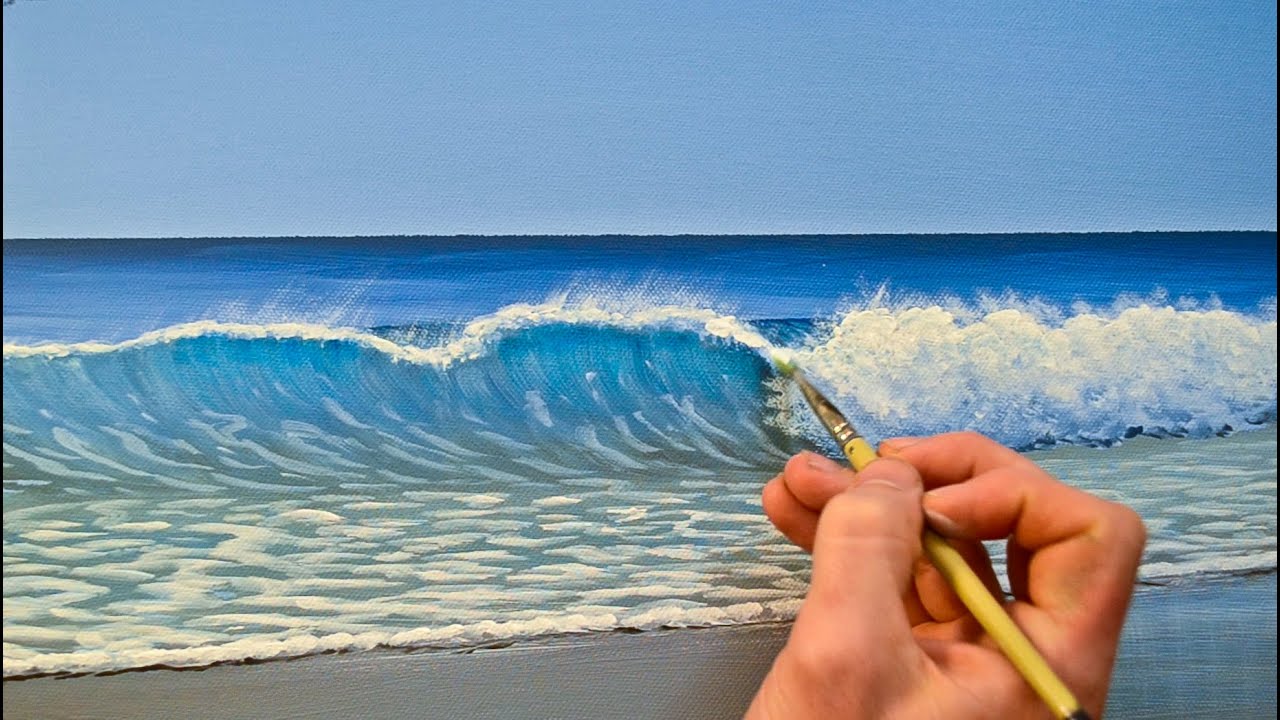The photograph captures an artist actively working on a nearly completed ocean scene painting that fills the entire frame. The artist’s right hand, holding a yellow paintbrush with white paint, is visible in the bottom right corner, meticulously adding details to the white foam of a breaking wave. The painting features a predominantly blue ocean with darker shades in the distance, transitioning to lighter blues as it approaches the foreground. A single wave with intricate foam patterns is just below a straight horizon line, situated about two-thirds up the canvas, meeting a clear blue sky. Below the wave, a small stretch of dull gray sand contrasts with the vibrant water above. The scene exudes a serene and detailed depiction of the ocean meeting the shore.